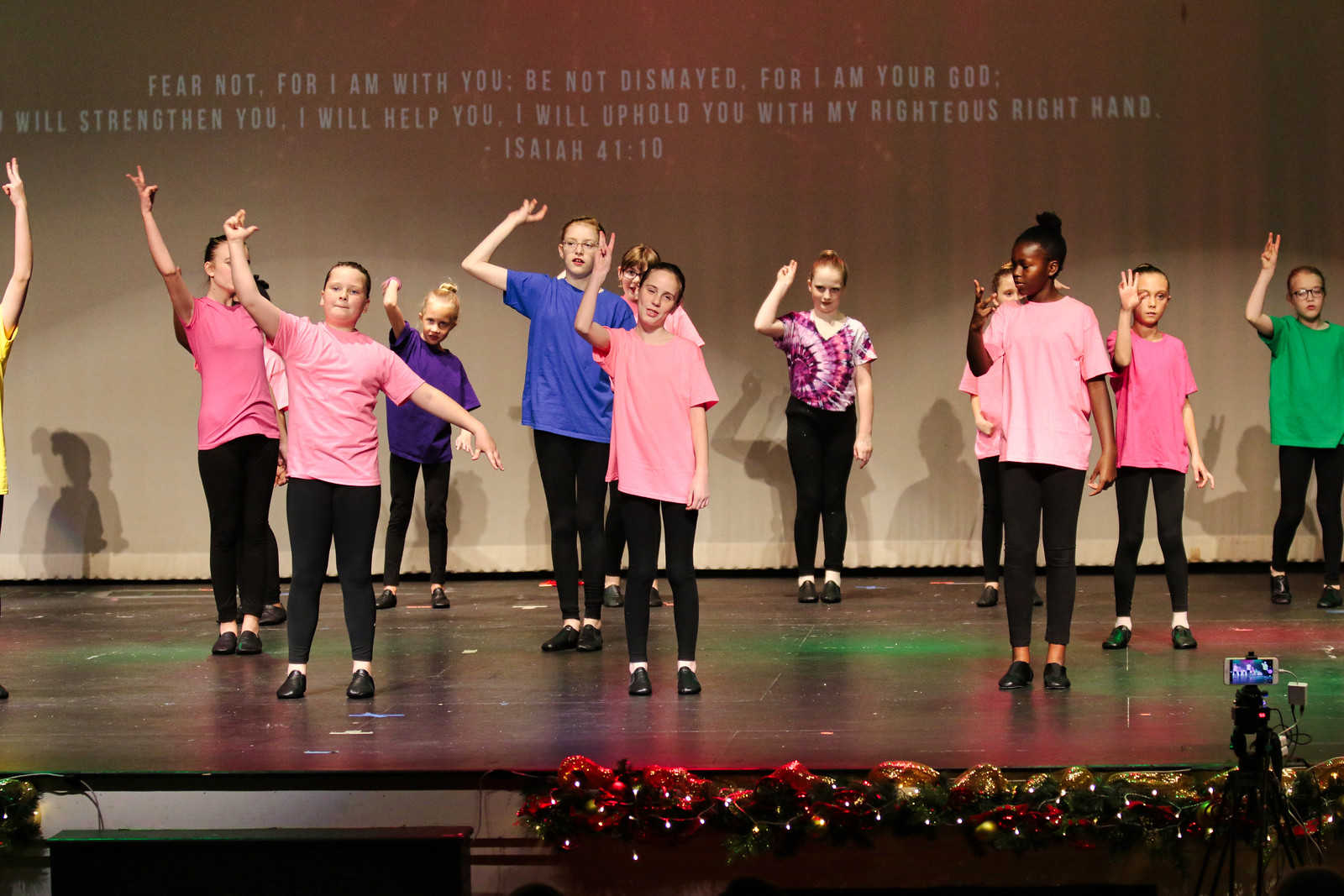A group of girls stands on a black stage floor, in front of a curtain backdrop with a projection that reads: "Fear not, for I am with you. Be not dismayed, for I am your God. I will strengthen you. I will help you. I will uphold you with my righteous right hand, Isaiah 41:10." The girls are uniformly dressed in black pants and black shoes, but their t-shirts vary in color: from right to left, they wear green, pink, pink, pink, tie-dye pink, blue, purple, pink, and pink. Each girl has her right hand extended in the air, facing the audience, which from our perspective appears as their left hand. They are making peace signs or claw gestures. Additionally, there is a phone set up on a tripod in the bottom left corner of the image, recording or taking a photo of the scene.